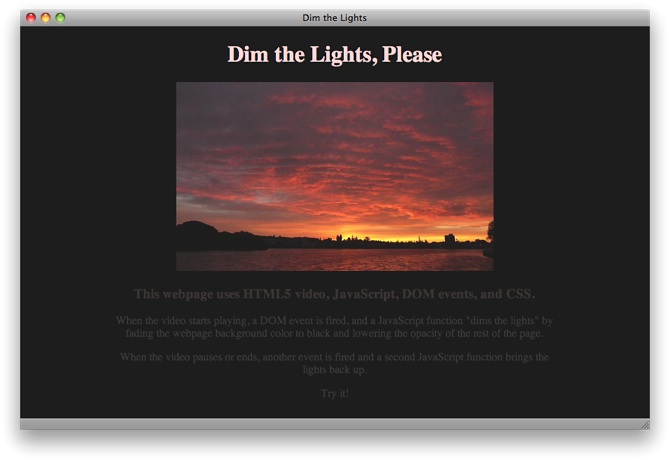A screen capture of a web page features a striking image of a sunrise or sunset in the center. The sky is awash with vibrant yellowish-orange hues, reflecting the natural beauty of the illuminated clouds in the upper half of the image. Above this colorful scene, white text reads, "Dim the lights, please." The background of the image is entirely black, creating a striking contrast.

Below the image, the page information clarifies that the website utilizes HTML5 video, JavaScript, DOM events, and CSS. An explanation follows, detailing that when the video begins to play, a DOM event triggers a JavaScript function designed to dim the lights by gradually changing the web page background color to black and lowering the opacity of the rest of the image. Conversely, when the video pauses or ends, another event triggers a second JavaScript function that restores the lights.

The explanatory text is challenging to read due to a choice of brown or gray font against the black background. This description appears to be a demonstration of how these JavaScript functions work in conjunction with HTML5 video and DOM events.